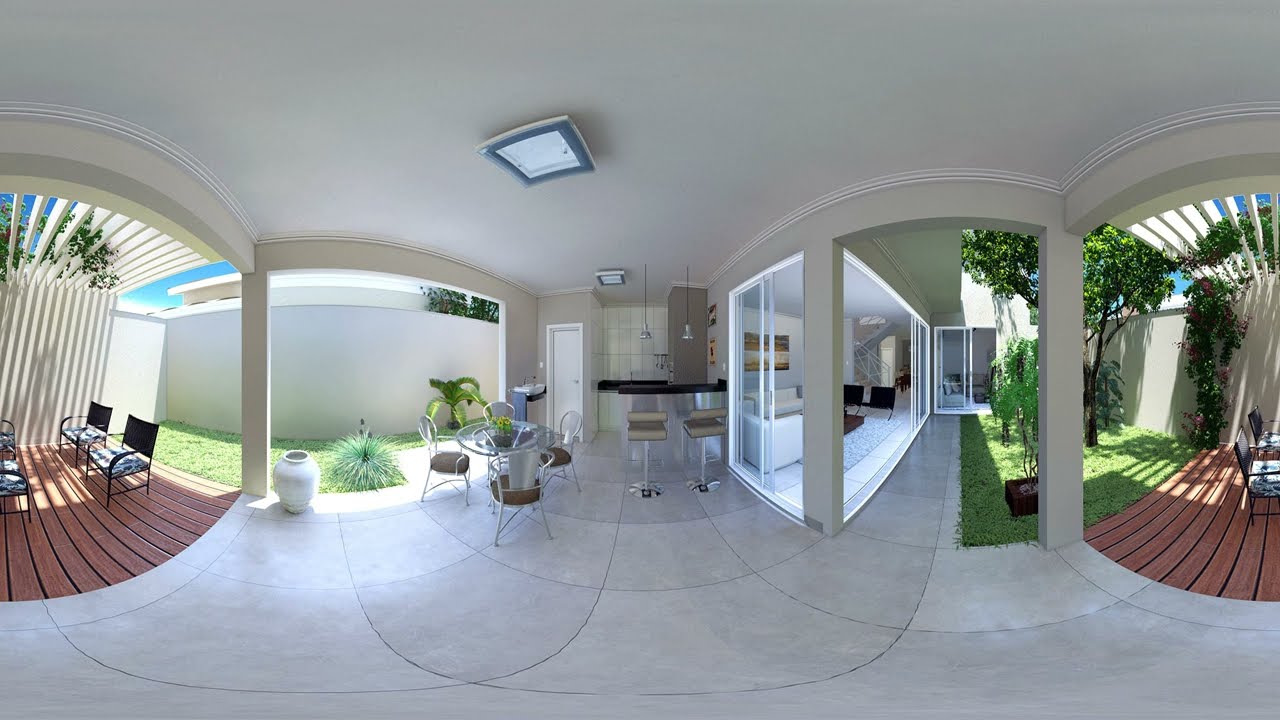The image appears to show a spacious and well-appointed backyard in a sunny region, possibly California or New Mexico. The foreground features a hard tile surface leading to an outdoor patio area. The covered patio has a white ceiling supported by white columns, with a white marble walkway directly in front. There is a modern outdoor bar with two sleek aluminum bar stools at the center, accompanied by a small circular table with three patio chairs.

Additionally, the yard includes two distinct patio areas. To the left, there's a circular table with three patio chairs and a small green lawn with some short outdoor plants and a sliver of blue sky visible. On the right, you can see red decking with black metal patio chairs and a vine climbing a white wall onto a trellis. This area also features a large tree with fanning branches.

Inside the home, visible through the backdoor entrance, there is a sunroom furnished with a white couch and fancy chairs. The interior walls display paintings, adding to the luxurious feel of the space. The outdoor area is equipped with cool lighting, a comfortable seating arrangement, and potentially a grilling area. The overall setting is bright, sunny, and richly landscaped, creating a relaxing and stylish atmosphere.